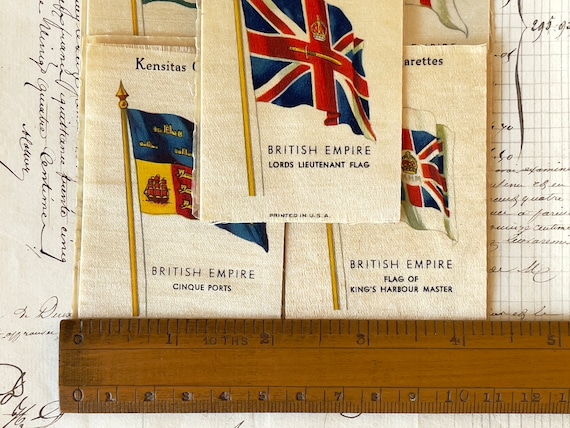This image captures a vintage collection of British Empire flags, likely intended for display or sale as historical memorabilia. Three primary fabric prints are arranged on a backdrop of old paper adorned with elegant, cursive writing, resembling calligraphy made with a quill. These prints each depict different flags of the British Empire, with their titles prominently marked below: "Lord's Lieutenant Flag" featuring the Union Jack, "Cinque Ports Flag," and "King's Harbour Master Flag." A wooden ruler, showing measurements up to 5 inches, is placed across the top of the prints, providing a sense of scale. The detailed craftsmanship of the flags and the historically styled background suggest the items are of significant vintage value, suitable for a museum collection.